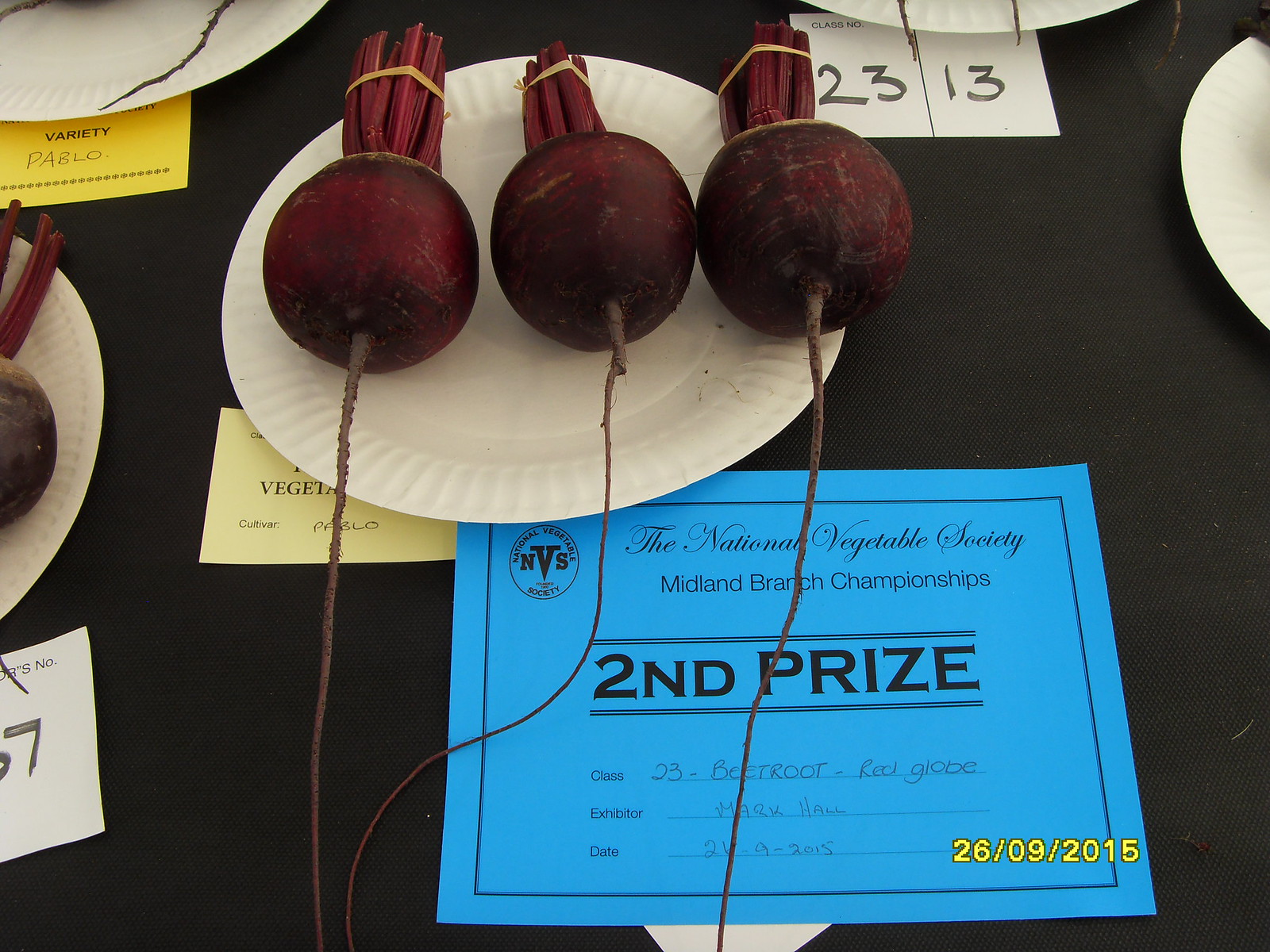In this color photograph, captured in landscape orientation, we are looking down on a table covered with a black woven tablecloth. Prominently in the center, there's a white paper plate situated towards the top with three large, perfectly round, dark red beets. These beets have lengthy single roots extending downward and their stems up above have been neatly cut off and tied with rubber bands. 

Beneath the plate, slightly to the right of center, lies a blue certificate with black outlines and print. This certificate is awarded by the National Vegetable Society Midland Branch Championships, proudly declaring "Second Prize." The lines below provide specific details with handwritten information: the class is noted as "23 Beetroot Red Globe," the exhibitor is "Mark Hall," and the date, confirmed by a yellow date stamp in the lower right corner of the image, is 26-09-2015. 

Surrounding the main focal point, the edges of other paper plates are just visible, suggesting an array of entries in this vegetable judging competition. The photo captures a moment of celebration in agricultural excellence, with the vivid colors of blue, yellow, and dark red standing out against the neutral background.